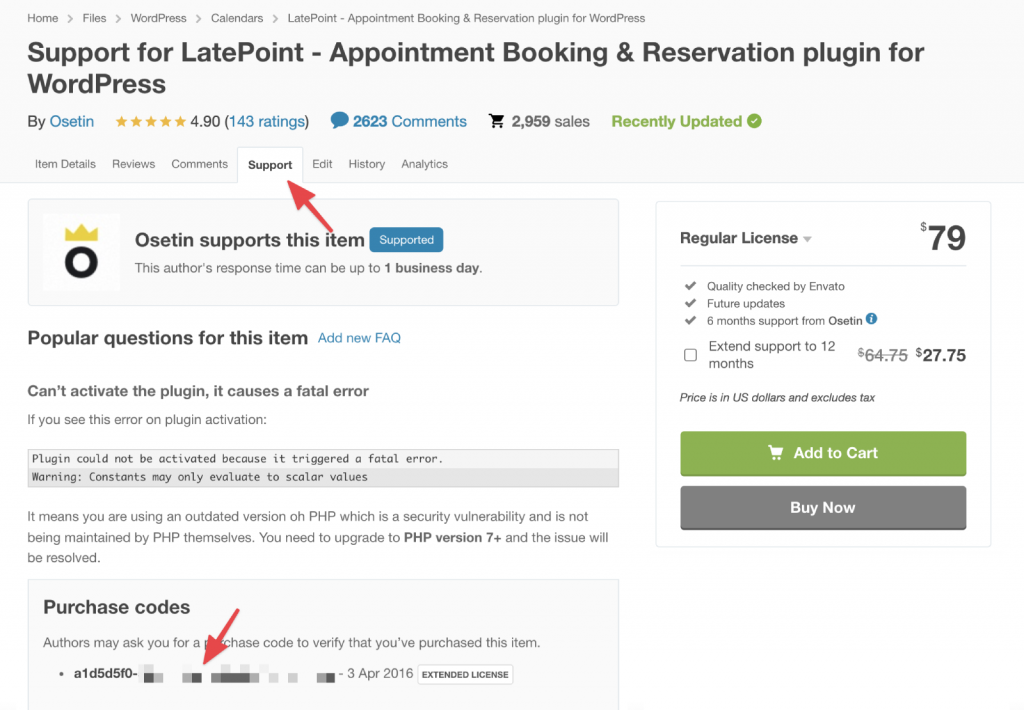The image depicts a detailed view of a WordPress page interface. At the top, the navigation menu includes the following options: Home, Files, WordPress, Calendars, Latepoint, and Appointment Booking and Reservation Plugin for WordPress. Below this menu, large text announces "Support for Latepoint, Appointment Booking and Reservation Plugin for WordPress by Ocedin". The page statistics show 2,623 comments and 2,959 sales.

Several tabs are present below the announcement, with the Support tab highlighted. A red arrow points to the highlighted Support tab, accompanied by the text "Ocedin supports this item. This author's response time can be up to one business day."

Further down, the section titled "Popular Questions for This Item" addresses common issues, such as the inability to activate the plugin due to a PHP fatal error. The resolution for this issue is upgrading to PHP version 7 or higher, as using outdated versions poses a security risk.

Another informational section titled "Purchase Codes" mentions that authors might request a purchase code to verify the purchase of the item.

On the right side of the page, a white background box displays the licensing options. The Regular License is priced at $79 and comes with benefits such as Quality Check by Envato, Future Updates, and Six Months Support from Ocedin. There's an option to extend support to 12 months for an additional $27.75, although this box is not checked. Below these options are the buttons "Add to Cart" and "Buy Now."